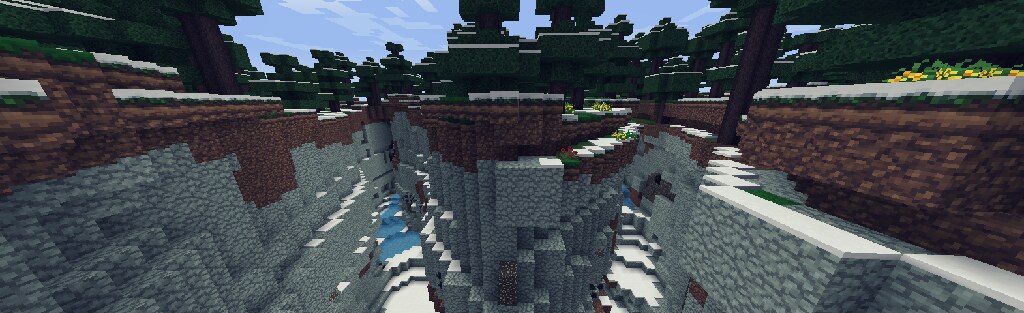In this captivating outdoor scene reminiscent of a video game, the world appears to be constructed from individual blocks of vibrant colors, adding a pixelated charm to the environment. Towering on either side of the scene are formidable walls; their lower sections are composed of gray stone, transitioning seamlessly into brickwork as they rise. Above, a cerulean blue sky features whimsically rectangular clouds, pieced together like an abstract mosaic of white. The sunlight bathes the scene, casting dynamic light and shadow across the various textures and surfaces. To the right, a splash of color is added by a cluster of vibrant yellow flowers perched atop a brick wall, contrasting against the structured austerity of their surroundings.